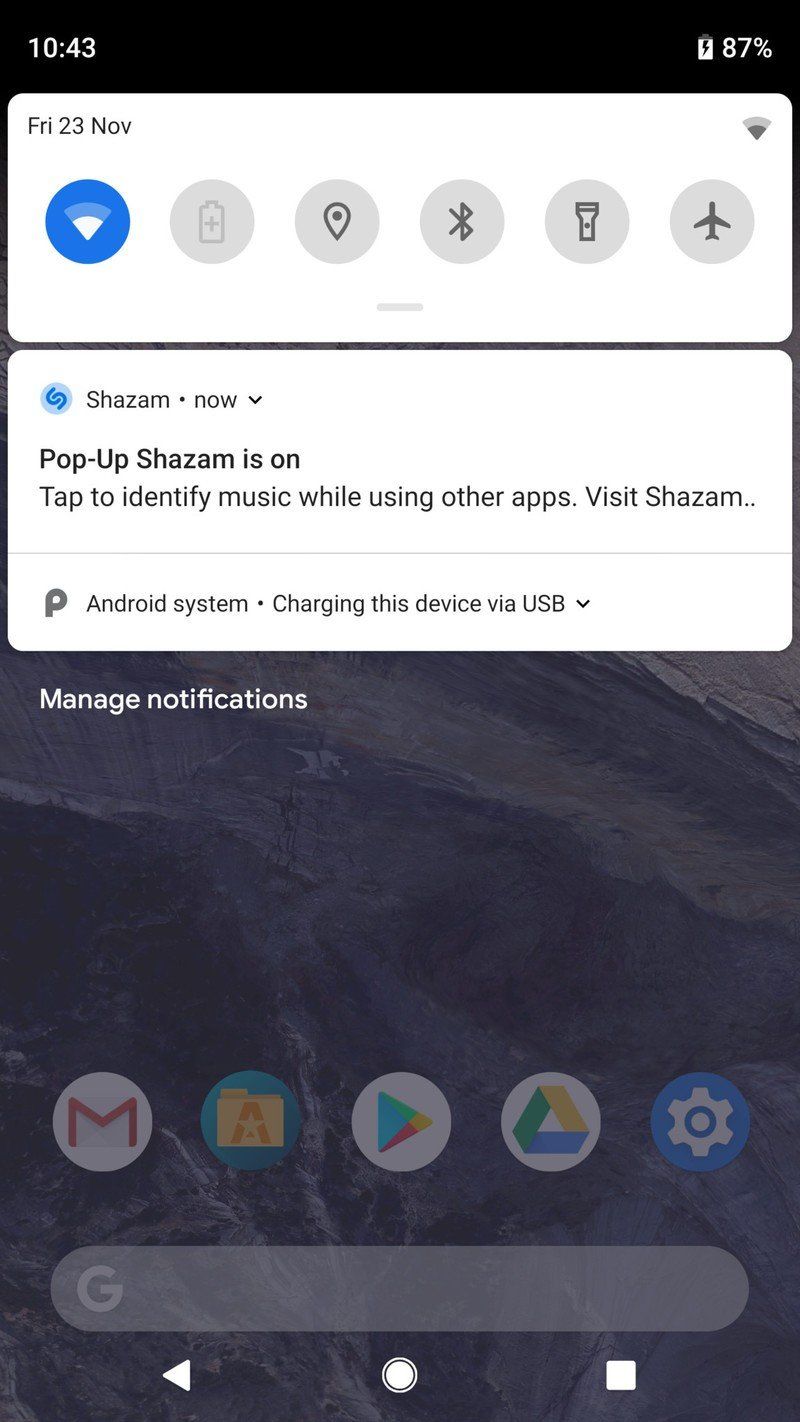Screenshot of a phone's notification bar captured at 10:43. The battery icon on the right indicates a charge level of 87%. Directly beneath the notification bar, a control menu shows the date as Friday, 23rd November. Several icons are visible in this menu: WiFi, Battery Saver, Location, Bluetooth, Flashlight, and Airplane Mode. The sole notification displayed is from Shazam, which indicates that pop-up Shazam is active. The notification reads: "Pop-up Shazam is on, tap to identify music while using other apps. Visit Shazam." The message is truncated by the notification window.